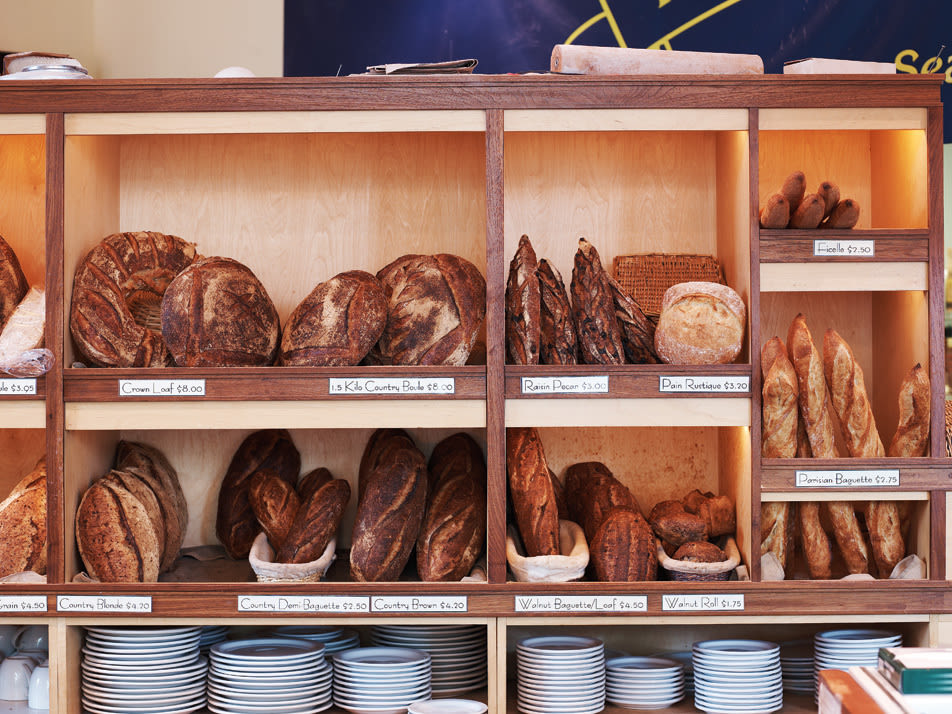The image depicts a detailed and meticulously arranged set of wooden shelves within a bread shop, showcasing an array of freshly baked bread types. The bottom shelf is stocked with various sizes of pristine white plates meant for customer use. Above this, a plethora of bread varieties is neatly organized on two main parallel shelves. The array includes country blend, country baguette, country brown, walnut baguette/loaf, and walnut rolls lined up side by side. On an upper shelf, there is a crown loaf, a cube country loaf, raisin pecan, and a pan roti. To the right, more baguettes transition upwards to a shelf that houses a ficelle bread. Adjacent cubicles contain additional items like parmesan baguette and unlabeled bread loaves, each marked with their respective prices. Behind the shelves, a large navy blue sign with an indiscernible yellow logo or writing hints at the shop's branding. This comprehensive display contrasts the warm browns of the bread with the clean white plates, embodying the inviting atmosphere of the bakery where customers can select their bread and enjoy a casual meal.